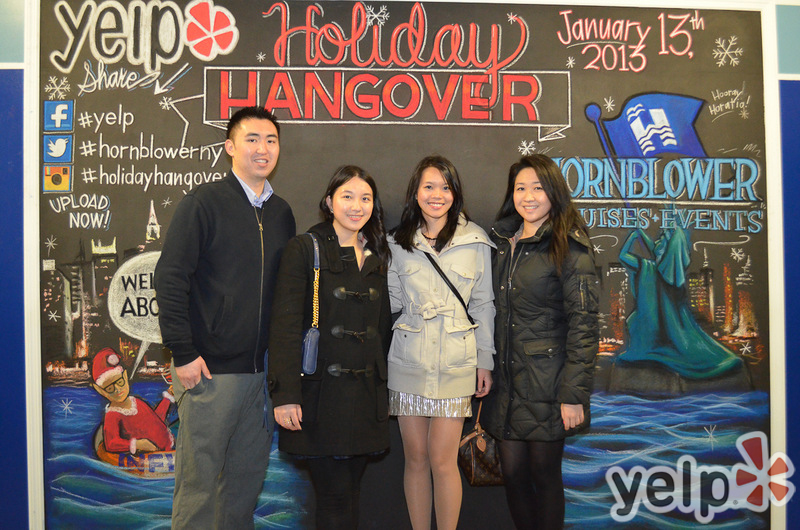The image features a group of four young individuals standing and smiling together in front of a detailed chalkboard backdrop. On the left stands a tall Asian young man with short black hair, wearing a black jacket and beige pants. Beside him is an Asian young woman with long black hair, dressed in a black coat. The third person in the line is another young woman with long black hair, wearing a white coat and a sparkly silver skirt. On the far right is a young woman with long black hair, sporting a thicker black coat. 

They are all positioned against a vibrant backdrop with a large "Yelp" sign displayed prominently in colorful letters, featuring red, blue, brown, and some creative elements like a snowflake dotting the 'i'. Above them, the handwritten chalk text reads "Holiday Hangover" in red script. To the right, the backdrop notes the event date, January 13, 2013, and features the Hornblower Cruises and Events logo with a distinctive blue flag and a stylized 'H'. The bottom left of the backdrop whimsically depicts an ocean scene with Santa Claus in an inner tube, accompanied by a speech balloon saying "Welcome aboard" and various social media icons. The overall atmosphere captured is one of festive celebration, likely at a party sponsored by Yelp, as indicated by the multiple appearances of the Yelp logo across the background.